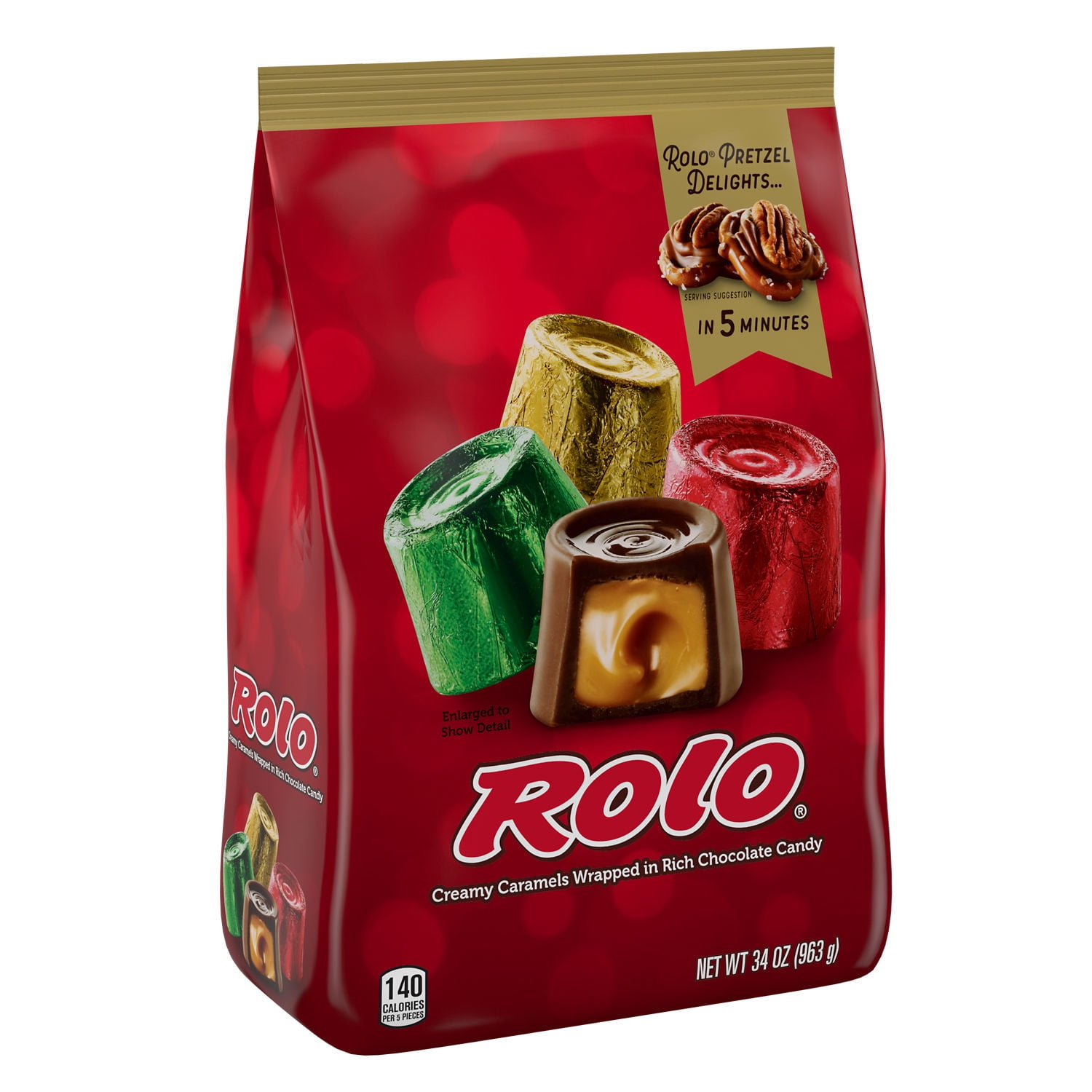The image depicts a detailed close-up of a vibrant red bag of Rolo candies, set against a pure white background. The bag tapers to a single edge at the top and features a gold seam. On the front, there is an image of four Rolo candies, three wrapped and one unwrapped with a bite taken out, revealing its creamy caramel center encased in rich chocolate. The candy is cylindrical, with the unwrapped one prominently displaying its luscious caramel interior. The brand name "ROLO" followed by a registered trademark symbol is prominently displayed, with the subtext reading "Creamy Caramels Wrapped in Rich Chocolate Candy." Additional text on the package reads "Rolo Pretzel Delights in five minutes," suggesting a recipe on the back for a quick, delectable treat. Other details on the front of the package include "140 calories" in a logo on the bottom left and the net weight of "34 ounces (963 grams)" on the bottom right. The overall aesthetic of the packaging, with its red, green, and gold colors, resembles a festively wrapped Christmas present.